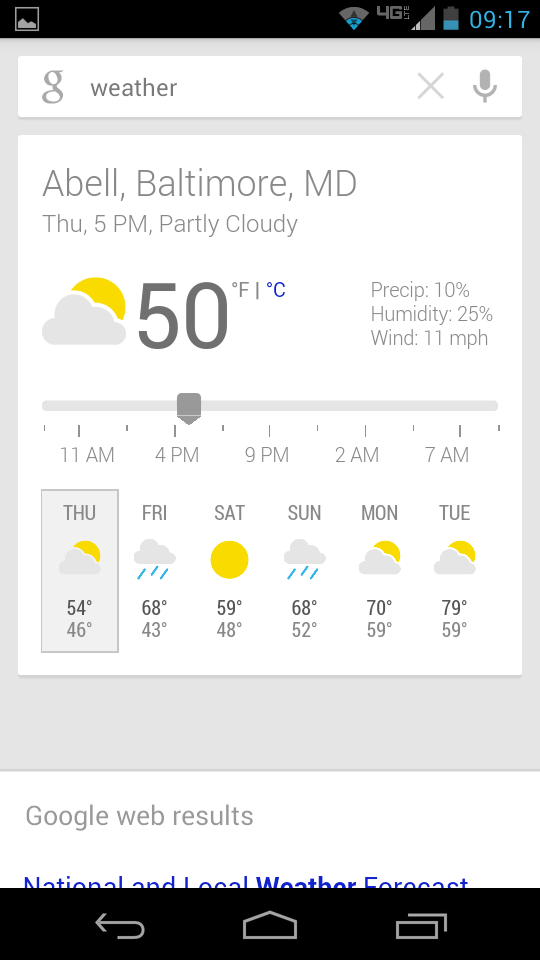Here is a cleaned-up and detailed caption for the image described:

---

Screenshot of a cell phone displaying a weather update in a mobile web browser:
- The top black border contains essential icons: 
  - On the left, there’s a grey image icon.
  - On the right, in blue, it displays "9:17".
  - The battery icon shows half full in blue with a grey top half.
  - The signal strength icon indicates one bar with "4G" next to it.
  - The WiFi icon also shows half strength, blue on the bottom half and grey on the top half.

- Below this, a light grey border holds a white search tab:
  - On the left, a grey "G" Google icon.
  - Next to it, "weather" is typed out.
  - On the right, a microphone icon and an "X" for clearing the search.

- Below the search tab, another light grey border leads to a white section containing weather information:
  - In the top left corner, it reads "Bell, Baltimore, MD."
  - Below that, "Thursday 5 PM" with a "partly cloudy" description.
  - An icon of a cloud with the sun peeking out on the right visually represents this.
  - The temperature shows "50°F."
  - On the right, details on precipitation, humidity, and wind are listed.

- A horizontal bar with a slider spans across indicating times:
  - Marked from "11 AM" to "7 AM," with intermediate times at "4 PM," "9 PM," and "2 AM."

- Below this bar is the weather forecast extending from Thursday through Tuesday.

- The bottom section outside the grey area:
  - In black, it reads "Google Web Research."
  - In blue, "National and local weather forecast."

- The very bottom features another black border with navigation icons in grey:
  - An arrow pointing up and to the right.
  - A back arrow pointing left.
  - A home icon.
  - A square with another overlapping square indicating open apps.

---